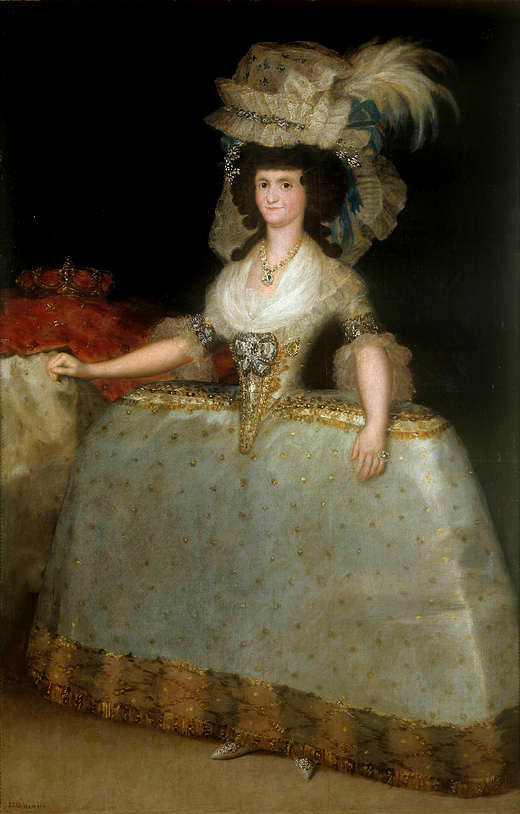The image portrays a white woman in a stylized medieval or possibly Elizabethan gown, characterized by its unusual shape—narrow from front to back but wide from side to side, reminiscent of traditional hoop skirts. The long gown extends to the floor, partially revealing her pointed shoes. She has a slightly heavy-set appearance by modern standards, with exposed, pasty arms extending from sleeves that reach her elbows. Her attire is predominantly in golden yellow, brown, and black hues.

Her dark, curly hair is adorned with a large, ornate, feathered hat, affixed above her head. She wears a gold necklace and additional jewelry, enhancing her regal appearance. The background is black, creating a stark contrast that emphasizes her figure. To her right (left from the viewer's perspective), a red object, possibly on a table, is visible. The woman gazes directly at the viewer with an unwavering, steady stare.